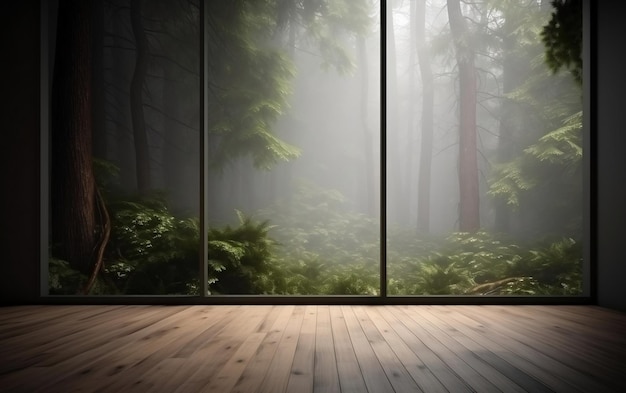The image depicts a digitally rendered, highly realistic indoor scene in landscape orientation, seamlessly blending details of a rustic but modern room and a lush, dense forest outside. The room features a slightly stained and polished wooden floor with highly visible grain on the planks, leading up to an expansive floor-to-ceiling, three-pane panoramic window that occupies almost three-quarters of the frame. This window, framed by narrow strips of wall on the right and left edges and punctuated by vertical metal frames, opens up to a misty, dimly lit forest teeming with lush green foliage and dense vegetation, including tall pine trees and thick ferns. The exterior appears to be captured at dusk, with faint sunlight piercing through the dense canopy, casting a serene glow. The overall ambiance hints at a tropical or subtropical setting. The scene inside is minimalistic, with no visible furniture, focusing solely on the intimate connection between the indoors and the verdant wilderness beyond.